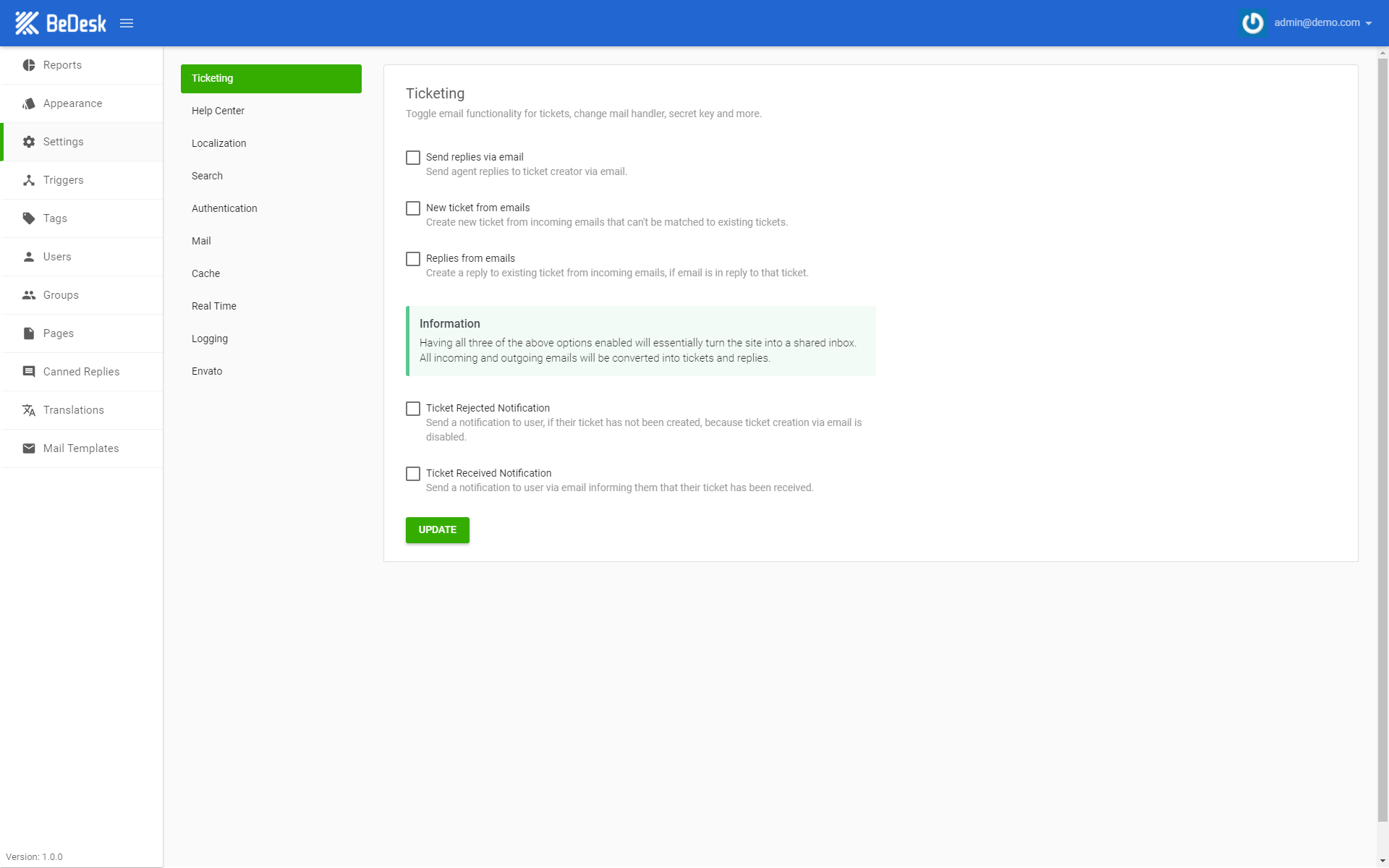**Detailed Caption:**

The image is a screenshot of a website with a variety of management features. In the top left corner, the site is branded with "B Desk" accompanied by a logo resembling lines forming a "K". Adjacent to the logo are three horizontal lines indicating a menu icon. The top right corner of the page displays the email "admin@demo.com" with a drop-down menu for selecting different accounts.

The page is organized into three sections. The far left sidebar features a navigation menu listing options such as Reports, Appearance, Settings, Triggers, Tags, Users, Groups, Pages, Can Replies, Translations, and Mail Templates. The "Settings" option is currently highlighted.

Consequently, the middle section displays sub-options under "Settings" that include Ticketing, Help Center, Localization, Search, Authentication, Mail, Cache, Real-Time Logging, and Envato. "Ticketing" is highlighted within these sub-options.

The rightmost section presents detailed settings for "Ticketing". Options include toggling email functionality for tickets, changing mail handlers, and configuring a secret key, each with a checkmark box for activation. Specific settings are listed:

- "Send replies via email": Send agent replies to the ticket creator via email.
- "New ticket from emails": Generate a new ticket from incoming emails that cannot be matched to existing tickets.
- "Replies from emails": Create a reply to an existing ticket from incoming emails that reference the ticket.

An information box explains that enabling all three options will essentially transform the site into a shared inbox where all incoming and outgoing emails are converted into tickets and replies. Additional settings include:

- "Ticket rejected notifications": Send a notification to the user if a ticket is not created because email-based ticket creation is disabled.
- "Ticket received notifications": Send a notification to the user via email informing them that their ticket has been received.

At the bottom of the settings, a prominent green "Update" button is visible for saving changes.